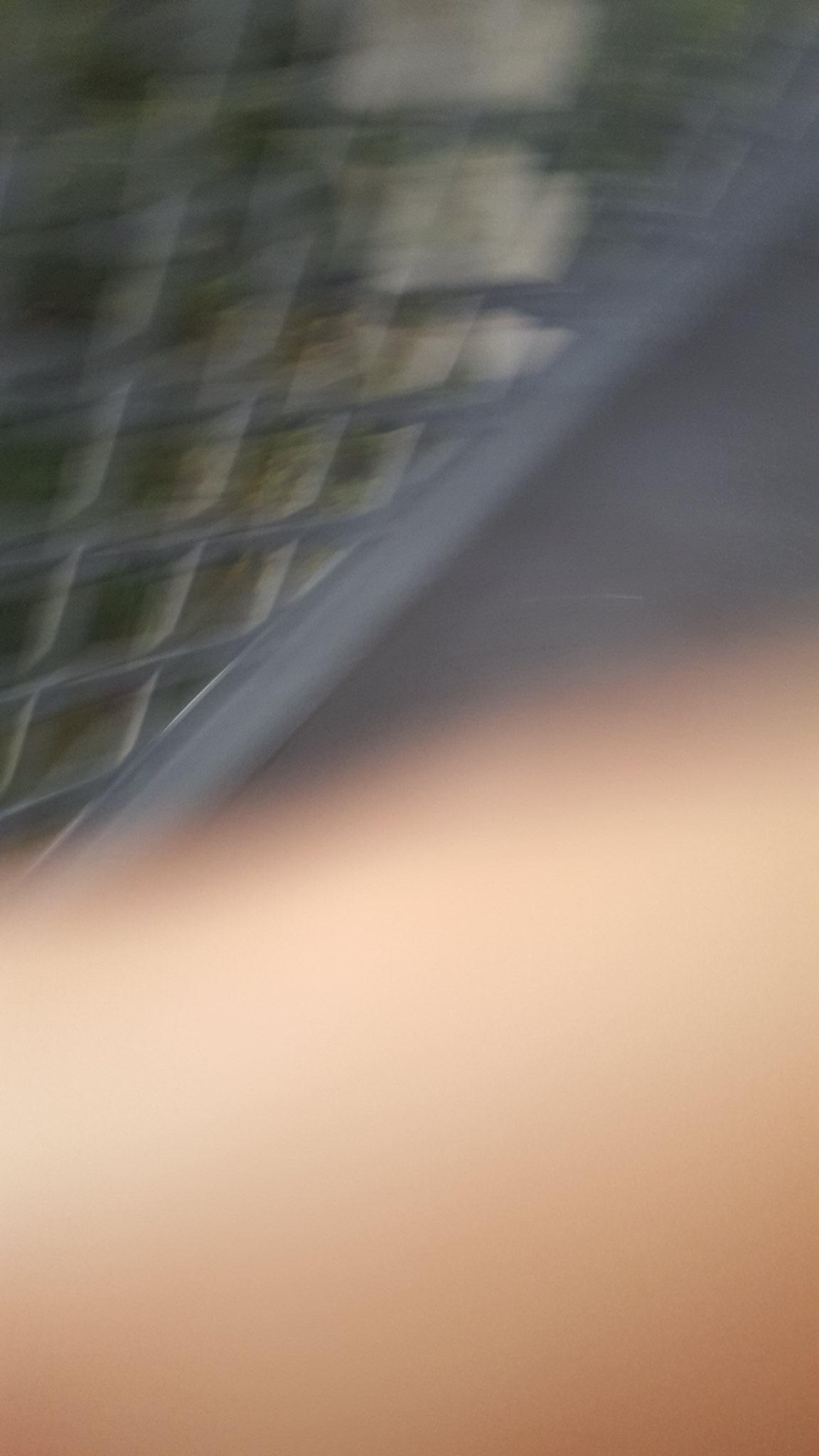The image is extremely blurry, taken outside in portrait mode with a part of a person's arm or finger, likely of a Caucasian individual, obscuring half of the frame. The background features a grey or white structure that could be a chain link fence or a garden trellis made out of wood, possibly indicating a balcony or deck. The ground appears to be a concrete or grey-colored walkway. Through the openings of the fence or trellis, there is visible greenery, likely trees or grass, adding a distant green contrast to the overall grey background. The overall scene is challenging to decipher due to the extreme blurriness of the photograph.